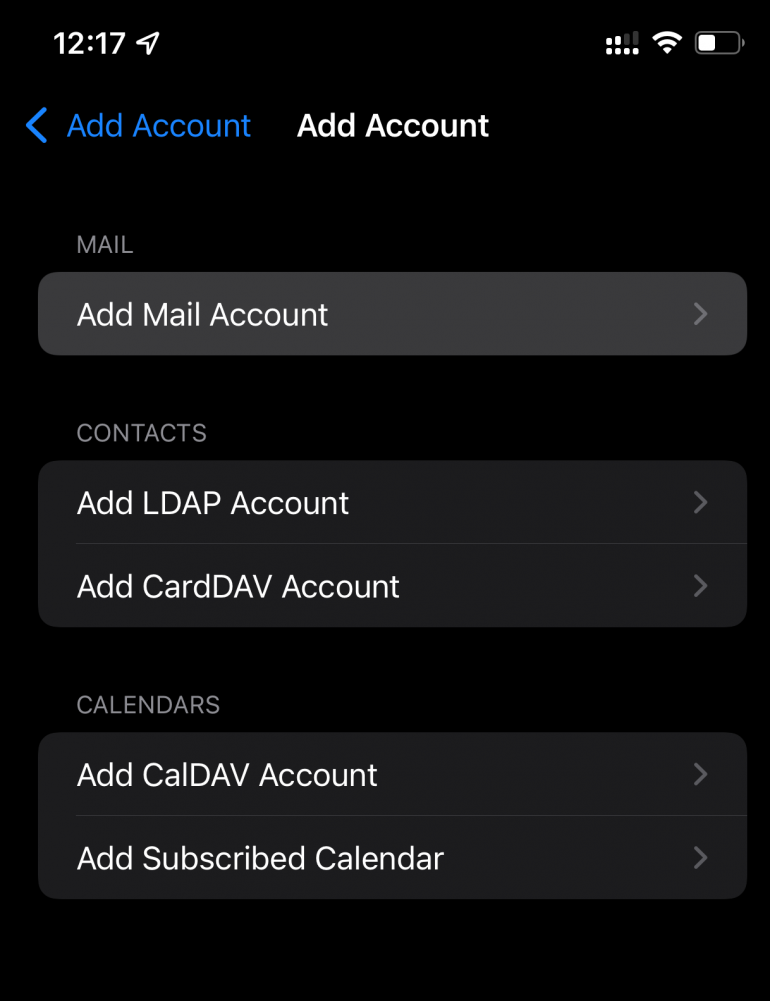The image depicts a smartphone settings screen, likely for an email application, featuring an account settings page. At the top, the screen displays the current time, "12:17," along with various icons indicating Wi-Fi connectivity and battery percentage. Dominating the center of the screen is a prominent blue "Add Account" button with white text that reads "Add account."

Below this, there are several sections listed:

1. **Mel**
   - Option: "Add Mel account"
   
2. **Contacts**
   - Option 1: "Add LDAP account"
   - Option 2: "Add CardDAV account"

3. **Calendars**
   - Option 1: "Add CalDAV account" (indicated with a gray arrow)
   - Option 2: "Add Subscribed Calendar" (also indicated with a gray arrow)

The text against the black background is mostly white and gray, enhancing readability, typical of a night mode setting. Most icons are white, maintaining the monochromatic aesthetic except for the blue "Add Account" button, which stands out.